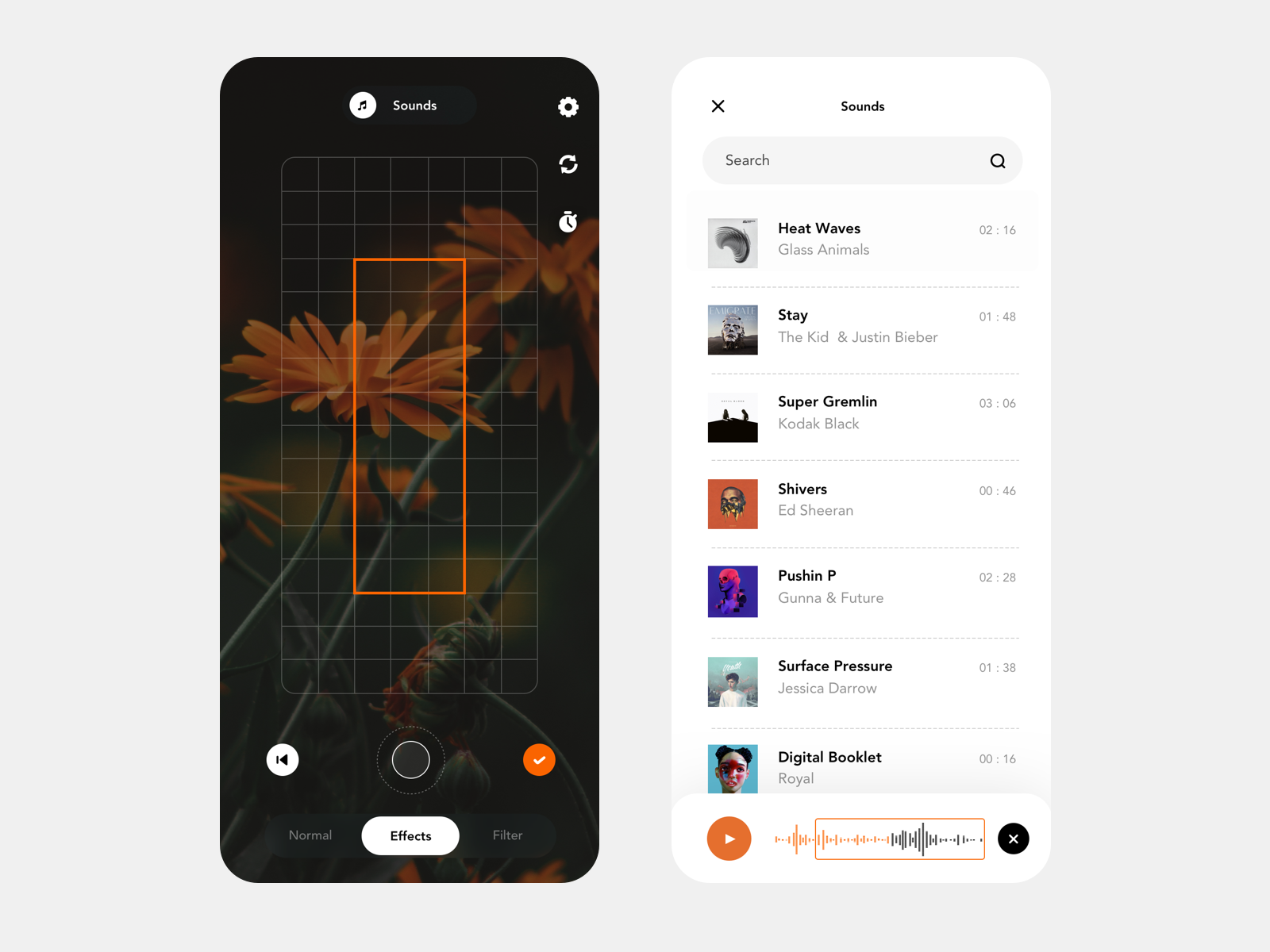This image showcases a side-by-side view of a smartphone interface, divided into two sections. On the left, the phone screen displays a camera interface with a black background. The screen features a gray grid pattern with an inner orange rectangle box. Overlaying the camera view are orange flowers with green stems. Along the bottom, there are interface options labeled "Normal," "Effects," and "Filter," with "Effects" highlighted. At the top of the screen, the word "Sounds" appears, and to the right, it displays icons for settings, undo, and a timer. Further down, between the "Normal" and "Effects" options, a back button, play button, and a red check mark icon with white contrast are visible.

On the right, the background is white, showcasing a playlist screen. At the top is a labeled "Sounds" section followed by a search bar. Below the search bar, a list of songs is displayed, including "Heat Waves" by Glass Animals, "Stay" by The Kid and Justin Bieber, "Super Gremlin" by Kodak Black, "Shivers" by Ed Sheeran, "Pushing P" by Gunna and Future, "Surface Pressure" by Jessica Darrow, and "Digital Booklet" by Royal. Each song title is paired with its respective album cover image on the left and a time indicator on the right. At the bottom of this section, there is a clipping tool intended for attaching music to the picture captured on the left side of the screen.